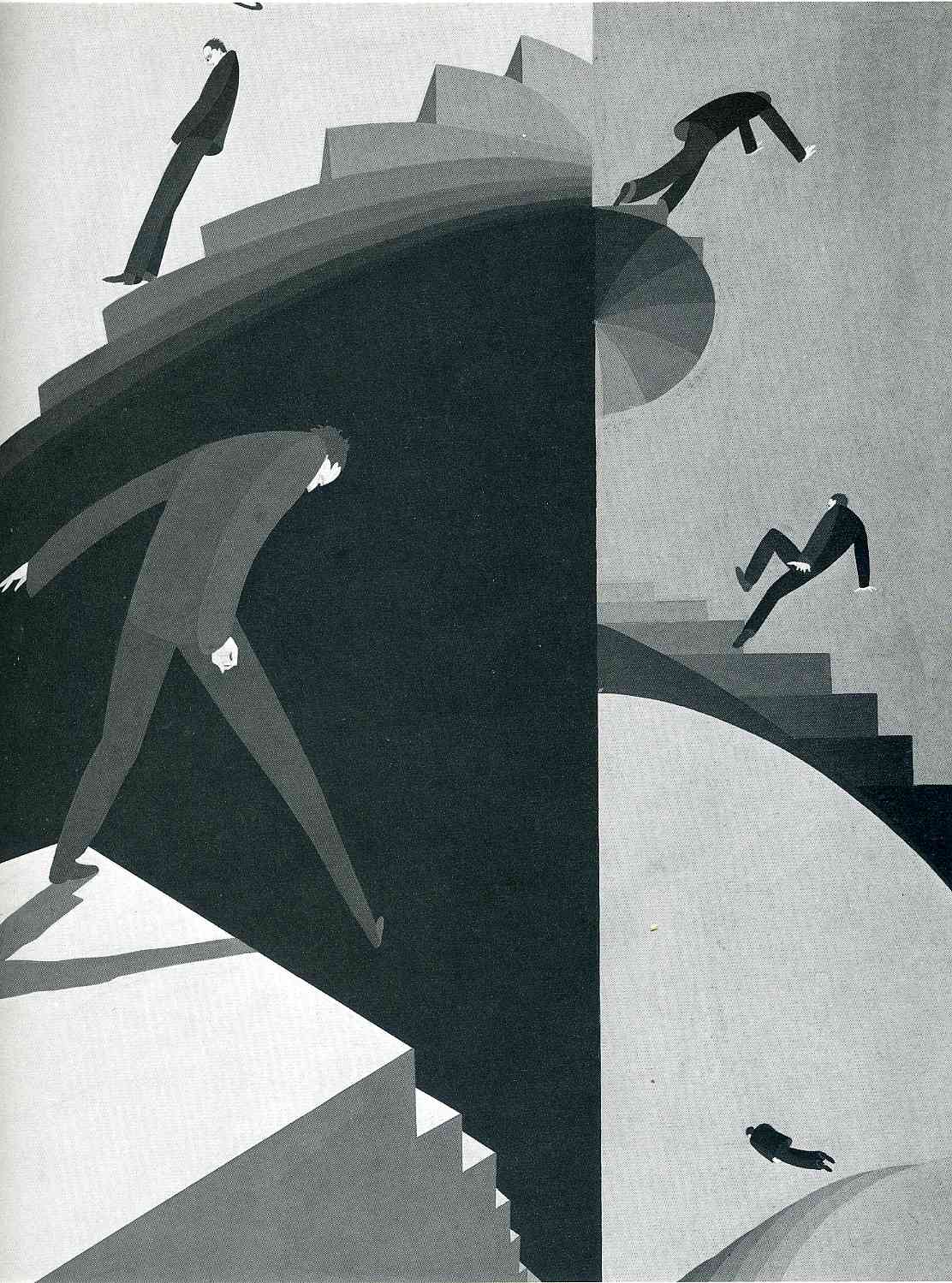The image is a surreal, MC Escher-esque illustration divided into two sections, featuring five elongated and exaggerated human figures interacting with various staircases. 

On the left side, at the top, there is a man in black with long legs and a small head looking down, standing straight on his heels beside a weird set of stairs. Beneath him, another man clad in dark attire descends steep, precarious stairs; his left foot is on the top platform, and his right foot dangles precariously. This section is set against a dark background that sharply contrasts with the figures.

In the thinner right section, the top features a man maneuvering down curving stairs that form a circular pattern. In the middle, another figure is climbing up stairs, his left leg bent as he leans backward with one arm behind him. At the bottom, the final depiction shows the man seemingly floating off a small hillside against a light gray background, giving an impression of detachment from the stairs altogether.

The overall image is surreal, with each depiction of the man appearing to navigate bizarre, abstract staircases, blending a dreamlike atmosphere with a sense of puzzling reality.